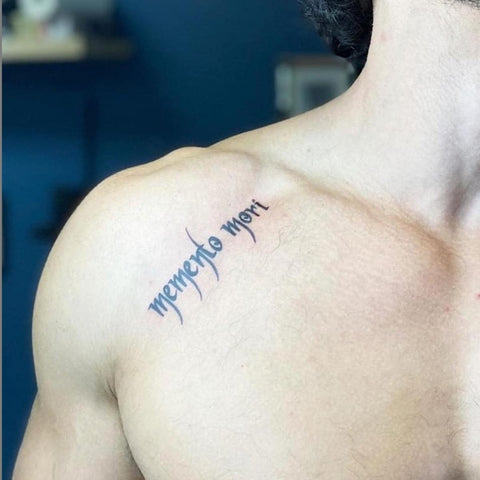The image features the left side of a shirtless man’s chest and neck. The focus is on a recently inked tattoo that reads "Memento Mori," written diagonally with black ink, stretching from the lower left towards the upper right, near the collarbone. The tattoo appears slightly reddish, indicating it is new. The man has long, black wavy hair visible at the top of the image but does not reach his shoulders. His bare shoulder and upper left bicep are visible, showing defined musculature and a glimpse of his clavicle. There’s also a hint of possible facial hair near the top right corner.